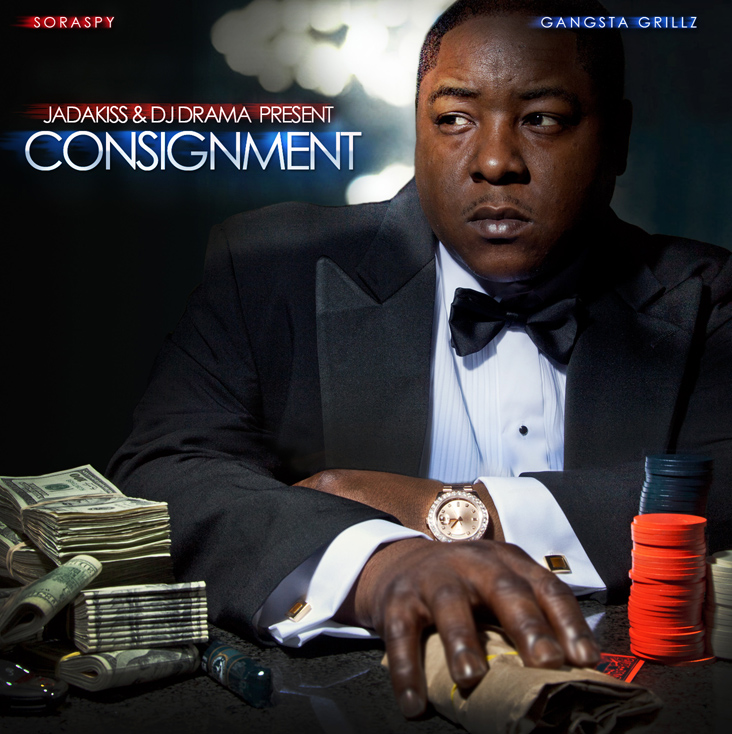The advertisement image features a distinguished man of African descent dressed in a classy black suit with a black bow tie and French cuffs. He exudes sophistication, accentuated by a fancy gold watch on his wrist. In his right hand, he holds a bag, while in front of him are wads of cash scattered to the left, and red and blue poker chips on the right, suggesting a casino setting. The background is predominantly black with faint lights, adding to the dramatic atmosphere. Prominent text on the left side reads "Jadakiss and DJ Drama present Consignment," while "Gangsta Grills" is displayed on the top right and "So Raspy" on the top left. The man's serious expression underscores the high-stakes ambiance of the scene.